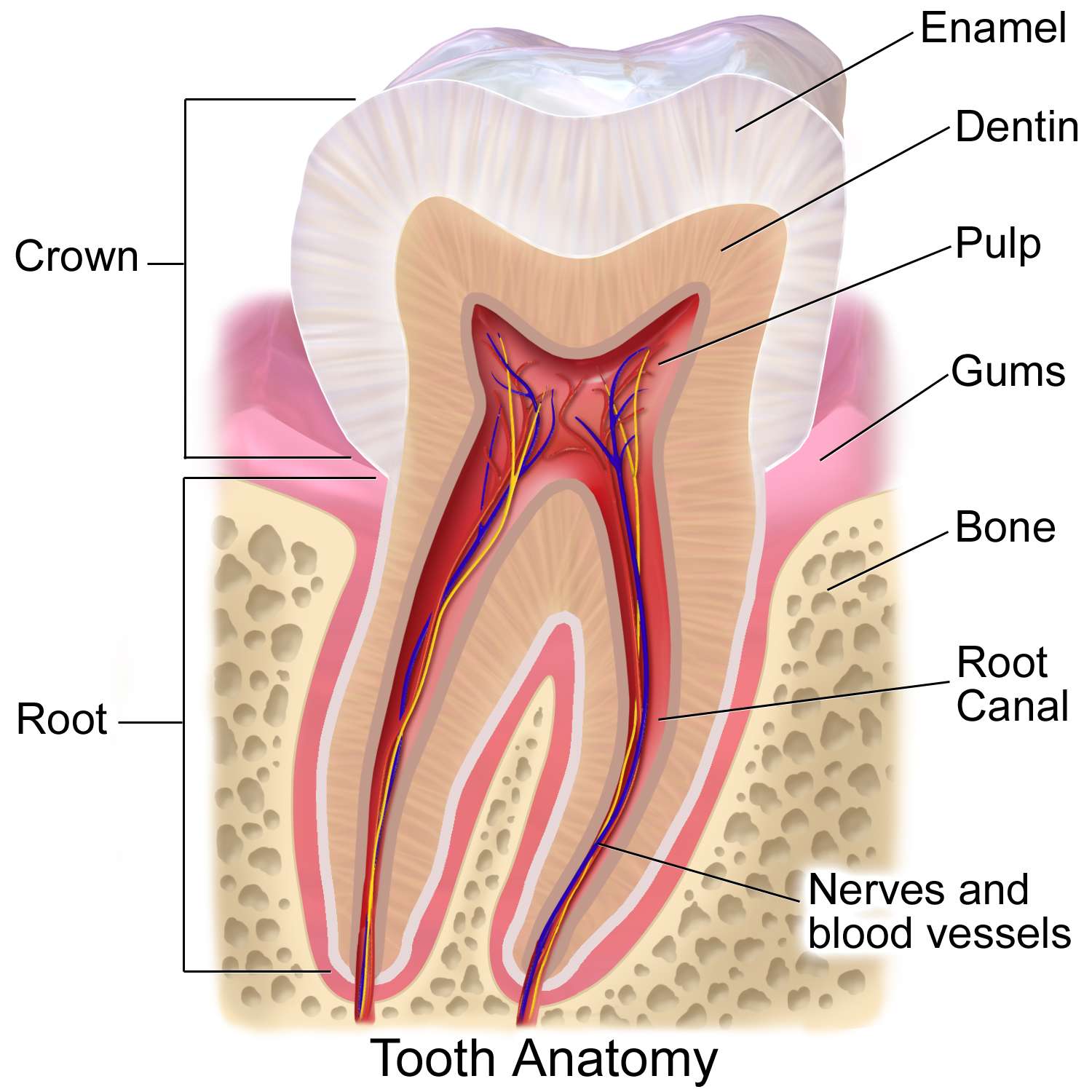The illustration is a detailed, labeled medical diagram of a human tooth, resembling those found in medical journals or textbooks. It features a cutaway view of a single molar, meticulously showing both the external and internal structures. The tooth is divided into two main sections: the visible upper part, known as the crown, which is white and labeled as enamel, and the lower section beneath the gum line, identified as the root. 

The diagram highlights various layers and components. The topmost white layer is labeled enamel, the next inner brown layer is called dentin, and the innermost pink section is the pulp. The area surrounding the tooth at the gum level is pink and labeled gums, with a brown textured surface identified as bone beneath it. The diagram also includes intricate details showing the interior of the root, where the root canal is located. This section contains small red, blue, and yellow lines representing nerves and blood vessels. The entire image is captioned as "tooth anatomy" at the bottom, providing a comprehensive overview of the tooth's structural and functional components.